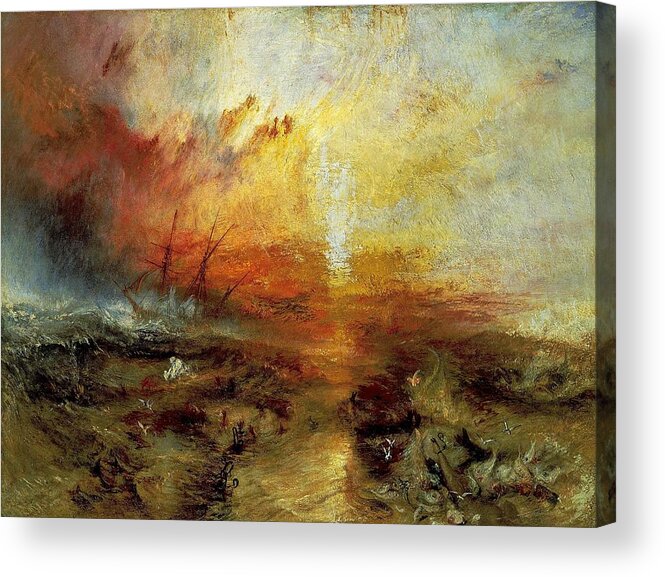This image is a detailed painting depicting an old-style sailing ship amid treacherous, choppy seas. The painting follows a wide vertical rectangle format, displayed on a canvas board that is angled slightly to the left, revealing its front and side edges with a white background. The scene conveys a sense of turmoil as the ship, centered towards the left, struggles against the formidable waves. The vessel, portrayed in rough condition with barely visible sails, is likely facing a life-threatening storm. 

The seascape at the bottom of the painting is heavily textured with murky, dark, muddy hues, indicating perilous waters. The sea is depicted in a range of dark browns, grays, and blacks, enhancing the stormy atmosphere. As the scene progresses upwards, the painting transitions into a brighter composition, with strong, directional sunlight piercing through the cloudy sky, predominating in the center and top regions. The left side remains darker, signifying the waning storm, while the right side brightens into an almost clear sky, possibly suggesting the storm's end or a false horizon.

The color palette used in the painting features an intricate blend of orange, yellow, gold, blue, white, gray, black, and green. These colors are used to manifest both the chaos of the elements below and the hope or impending calm suggested by the light above. The visual effect is amplified by the blurred, oily appearance of the brushstrokes, which create a sense of looking through a smeared lens, adding to the drama and intensity of the scene.